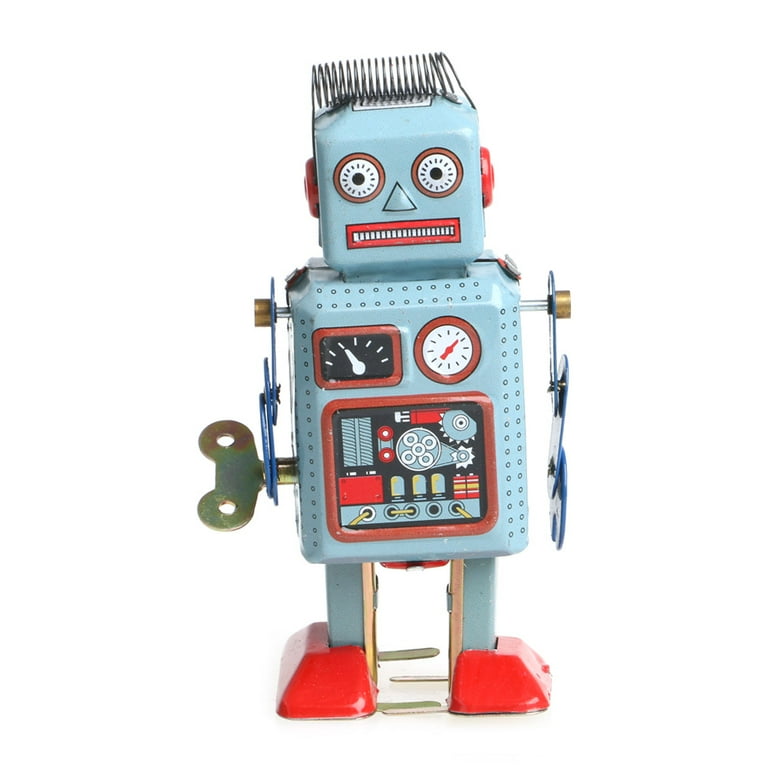This image is a detailed digital photograph of a vintage child's wind-up toy robot. The robot, primarily made of tin, features a box-shaped body and head, both painted in a baby blue hue. Prominently placed on the robot’s right side is a key crank used for winding it up. The robot stands upright on vibrant red shoes and has a pair of arms that likely flail when it moves. Its face boasts two circular eyes, a triangular nose, and a red rectangle for lips detailed with lines to resemble teeth. 

The front of the robot is adorned with a series of dials and gauges, adding to its mechanical charm. One gauge shows a white needle against a black background, while another round gauge features a red needle and tick marks. Further down, a small window reveals a glimpse of the robot's inner workings, including what appears to be vacuum tubes, gears, a battery, and various other components. Red rims accentuate the gauges and window, adding a pop of color to the blue and silver body. Bronze and yellow details are also visible, contributing to the robot's retro aesthetic. A spring-like coil reminiscent of a shock absorber crowns the top of the robot’s head, adding a whimsical touch.

The robot is positioned on a white surface with a white background, and the light source comes from the right side, casting soft shadows that enhance the overall clarity of the photograph.